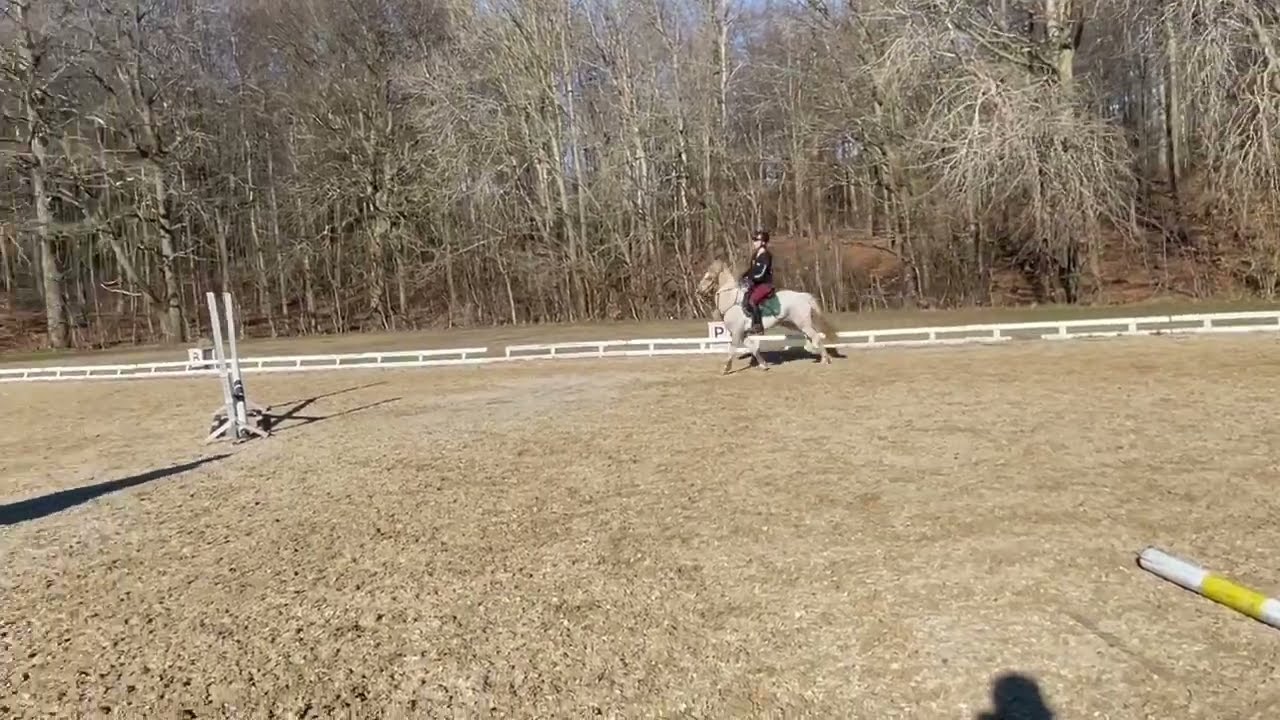In this photograph, a woman dressed in a black jacket and maroon pants, wearing a black helmet, is seen riding a large white horse. The scene is set on a fenced outdoor horse racing field, where the ground is a mixture of dry, beige grass and brown soil, indicative of fall or early spring. The white fence encircles the entire perimeter of the track, amid which various horse racing instruments are placed. On the left, two white poles with a shadowed X between them suggest a jumping obstacle. Stretching beyond the fence, the landscape features barren trees without leaves, adding to the chilly atmosphere captured under the morning sunlight, which casts clear shadows across the scene.